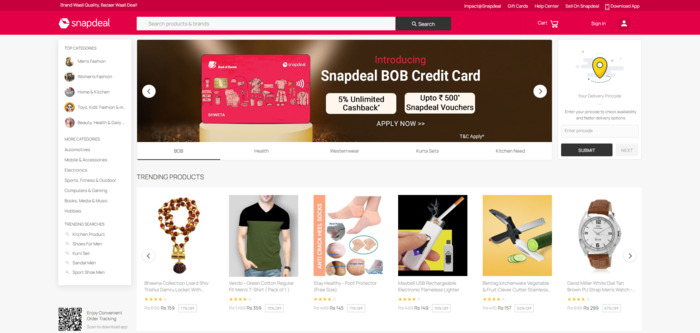The image is a screenshot of the Snapdeal website homepage. At the top-left corner, the Snapdeal logo is prominently displayed. Adjacent to the logo on the right is a search bar. Dominating the central area of the page is a promotional banner for the Snapdeal BOP credit card, featuring two buttons. The button on the left highlights "5% Unlimited Cash Back," while the button on the right offers "Up to 500 Snapdeal Vouchers." Below this banner, a series of product listings are arranged in a grid format. The first product appears to be an elegant necklace, followed by a stylish shirt, a pair of socks, a multi-functional knife, a sleek wristwatch, and a high-quality lighter.